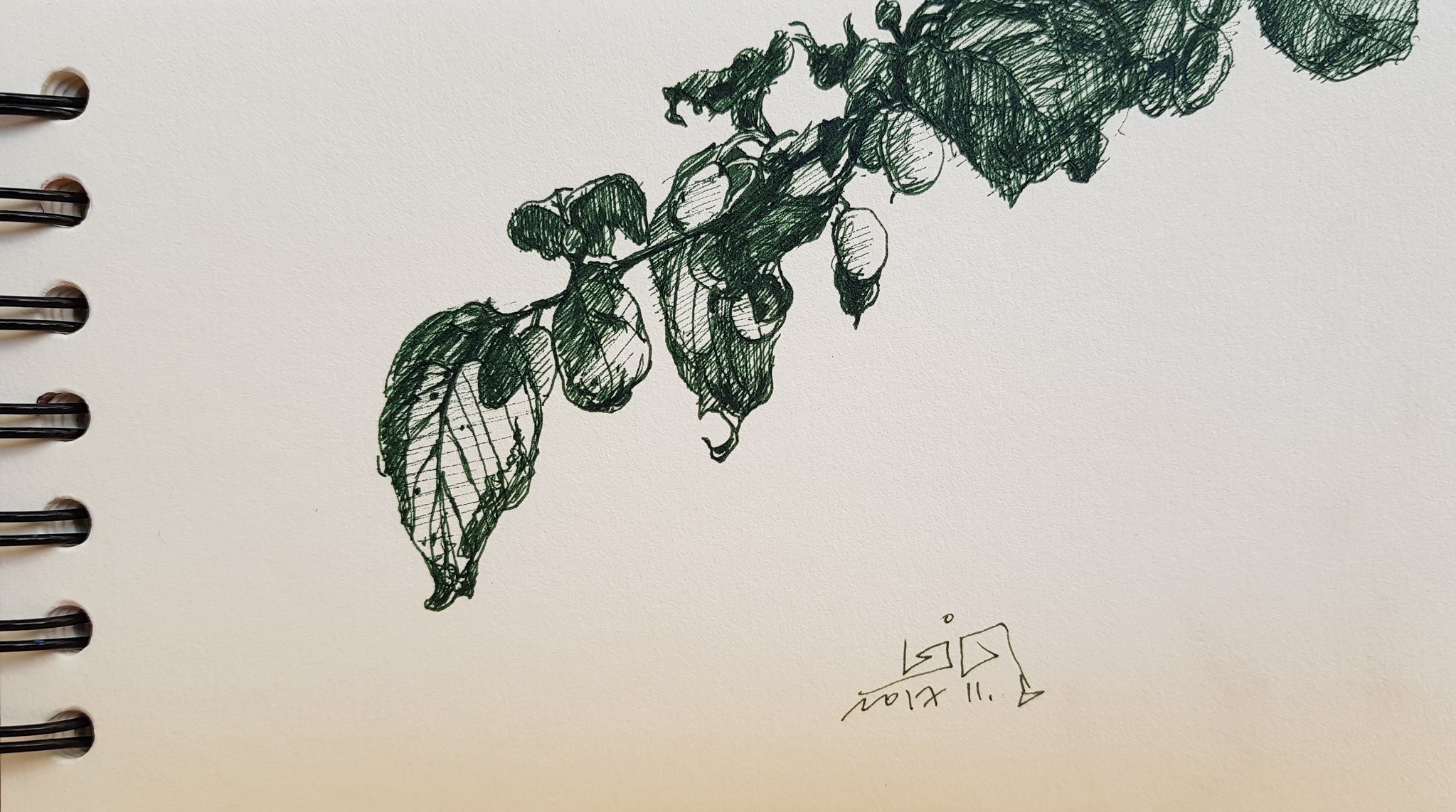This image showcases a detailed pen drawing on a notebook page. The notebook is characterized by its circular, vertical holes along the left-hand side, designed for spiral binding. A glimpse of the metal wire spiral binding is visible, with only two wire ends emerging from the circles. The drawing features an intricately detailed branch adorned with leaves and small berries. The veins in the leaves and careful pen strokes provide depth and shading to the illustration. A signature, though unreadable, is inscribed at the bottom of the drawing, indicating the artist's mark.